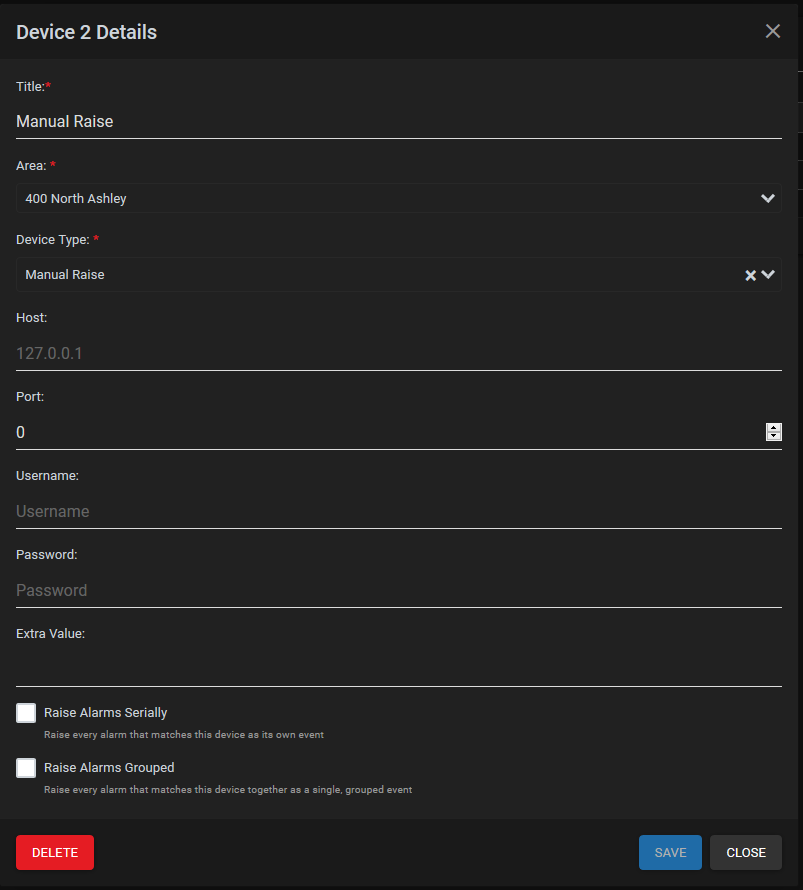This image displays a screen of a device interface, set against a black background. At the top of the screen, the text "Device Details" is prominently displayed. Below this, there is a section header titled "Title," marked with a red dot, followed by the text "Manual Raise." This section is separated by a white line stretching across the screen.

Beneath this division, there is another header labeled "Area," accompanied by a red dot. The text next to it reads "400 North Ashley." Following this, there's a section titled "Device Type," also marked with a red dot, displaying the text "Manual Raise." Below this, under the label "Host," someone has entered "127.0.0.1," shown in gray text.

Continuing downward, the label "Port" is followed by a colon and the number "0." Another white line separates this from the next section. The following sections display "Username:" and "Password:" with the corresponding placeholder text "Username" and "Password" in gray. Beneath these is another section labeled "Extra Value," with a white line and no provided input.

At the bottom of the screen, there are two buttons: a "Delete" button located in the bottom-left corner and a "Save and Close" button on the bottom-right corner.